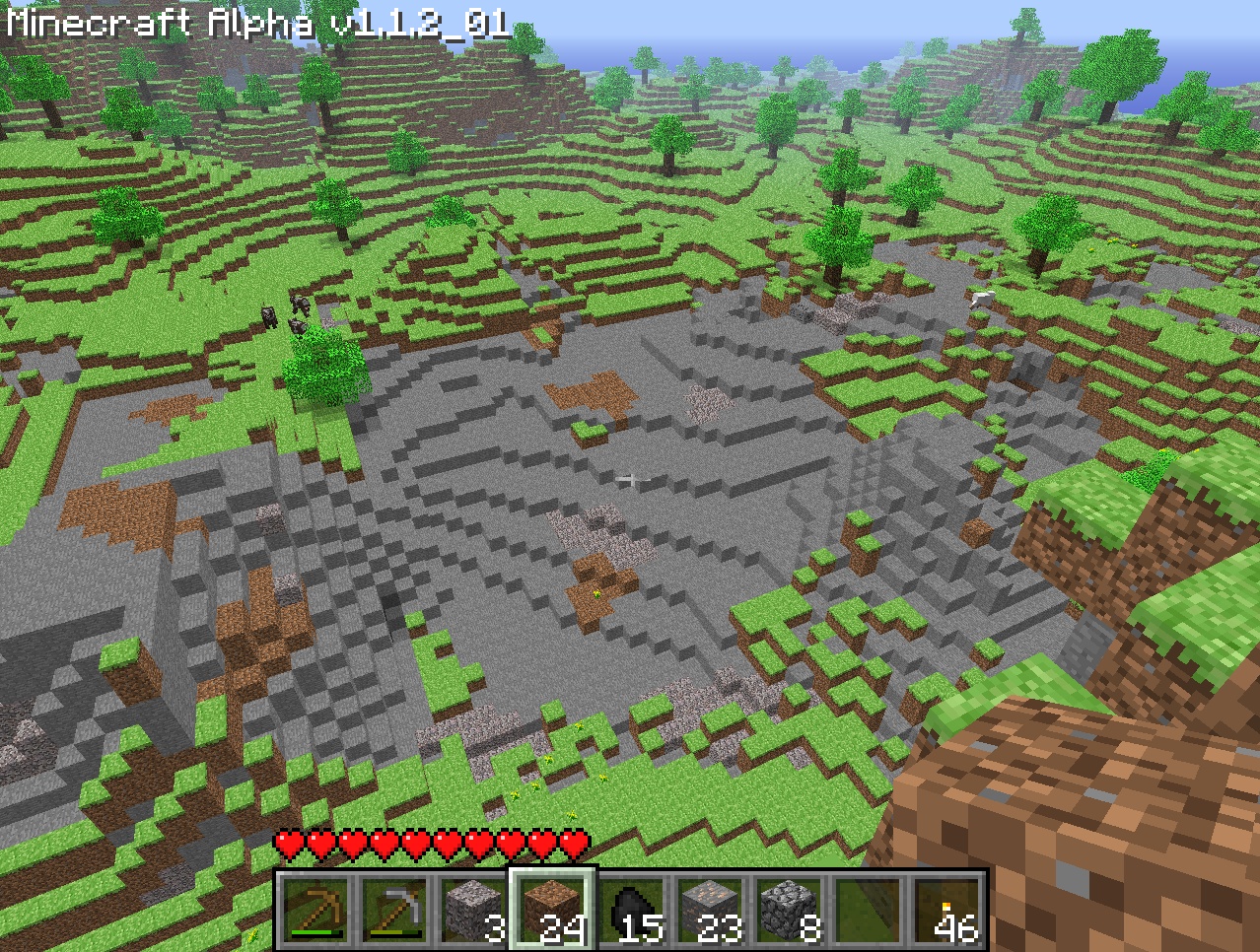This color photo captures a screen from the game Minecraft, specifically denoted as "Minecraft Alpha v 1.1.2_01" in white, pixelated text at the top left corner. The image shows a pixelated, cubic terrain resembling a Lego-like construction, characterized by a mix of gray, brown, and green elements. The landscape predominantly features stone and gravel, transitioning into grassy and hilly areas dotted with various dark green trees. In the distance, a cow can be vaguely seen. The player's interface at the bottom includes several tools and blocks with quantities displayed beneath them, and a row of ten red hearts above. The player appears to be holding a dirt block, contributing to a typical, yet vividly detailed Minecraft scene.